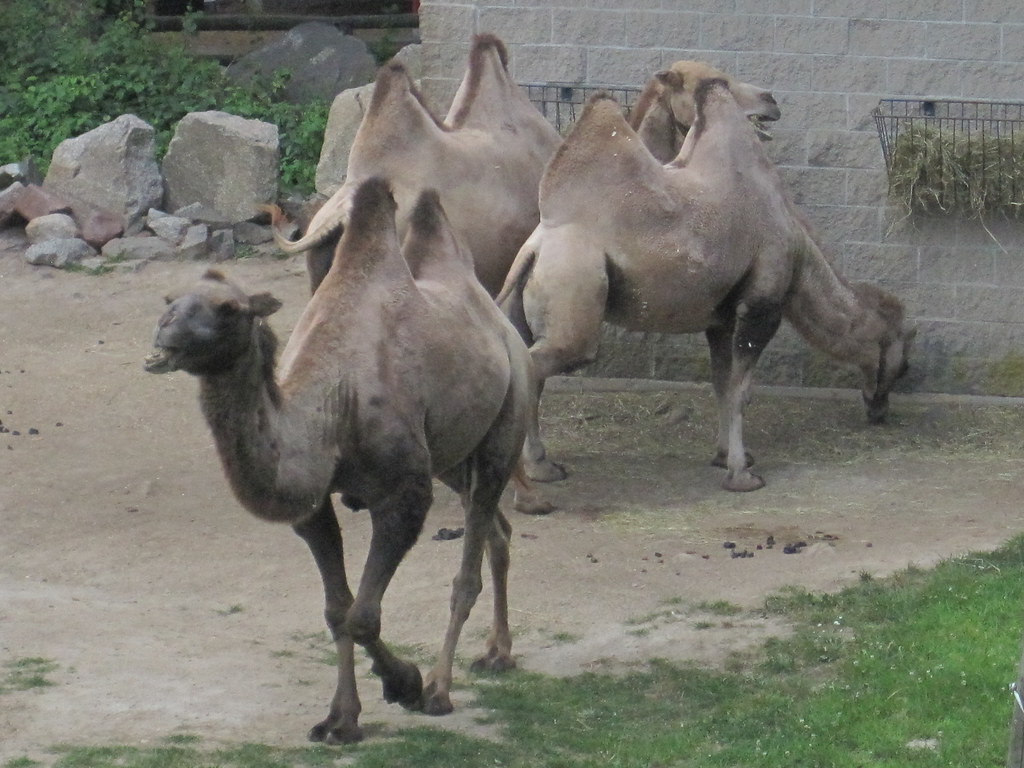This detailed, scenic outdoor photograph showcases three brown, two-humped camels, likely enclosed within a zoological exhibit. The foreground features a single camel standing on sandy, light brown soil, with one leg poised as if to walk, its face angled slightly away from the camera. The area immediately surrounding the camels is mostly barren save for a small patch of grass situated in the bottom right corner. Further back, two camels have their backs turned to the camera; one is bending down, seemingly to eat from the ground. The background is marked by a grey stone wall adorned with hay feeders, indicating the potential zoo setting. Beyond the wall, additional natural elements such as rocks and sparse shrubbery are visible, adding depth and context to the image of these majestic animals.